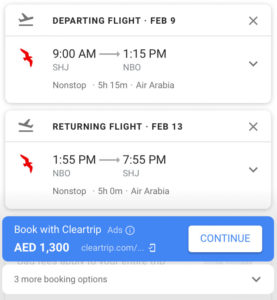The screen displays a detailed itinerary for an upcoming flight. The information is organized into two main sections, each delineated by distinct colored boxes—blue for departure and white for return.

In the left section, labeled "Departing," there's a small graphic of a plane taking off. Additionally, a red bird icon whimsically flies across the time frame, adding a humorous touch. The departing flight is scheduled for February 9th, with a takeoff at 9:00 a.m. and arrival at 1:15 p.m., flying non-stop from SHU to NBO on Air Arabia. The total journey time is 5 hours and 15 minutes.

The right section, labeled "Returning," mirrors the departure format. Here, another plane graphic indicates the return flight, with another amusing red bird icon hovering over the time. The return flight is on February 13th, departing at 1:55 p.m. and landing at 7:55 p.m., also non-stop from NBO back to SHU on Air Arabia. This leg of the trip takes 5 hours.

Additional information indicates that the flights can be booked through Cleartrip.